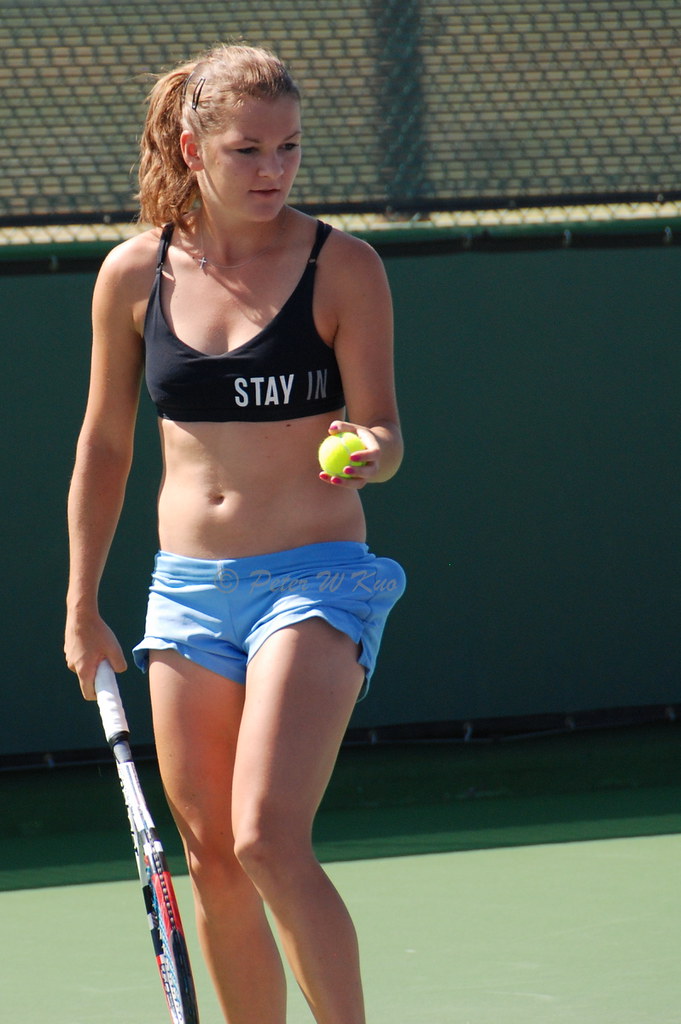The photograph captures a close-up scene of a young white female tennis player in an outdoor setting. She is facing to the right and stands on a green tennis court, partially enclosed by metal railings visible in the background. Her light brown hair is neatly tied back in a ponytail, adorned with a few visible barrettes on the right side. She is dressed in a small black sports top with “STAY IN” written in white uppercase letters on the lower corner, paired with very small light blue shorts that sit about four inches below her belly button, exposing her midriff.

The woman wears a silver chain necklace with a small silver cross pendant. In her right hand, she holds a tennis racket with a white grip and red and black accents, positioned downwards toward the ground. Her left hand holds a tennis ball, and her fingernails are painted with red nail polish. Another tennis ball seems to be in the pocket of her shorts. The photograph is vertically oriented and cuts off at her feet, with a copyright superimposed on her shorts reading "© Peter W. Kuo."